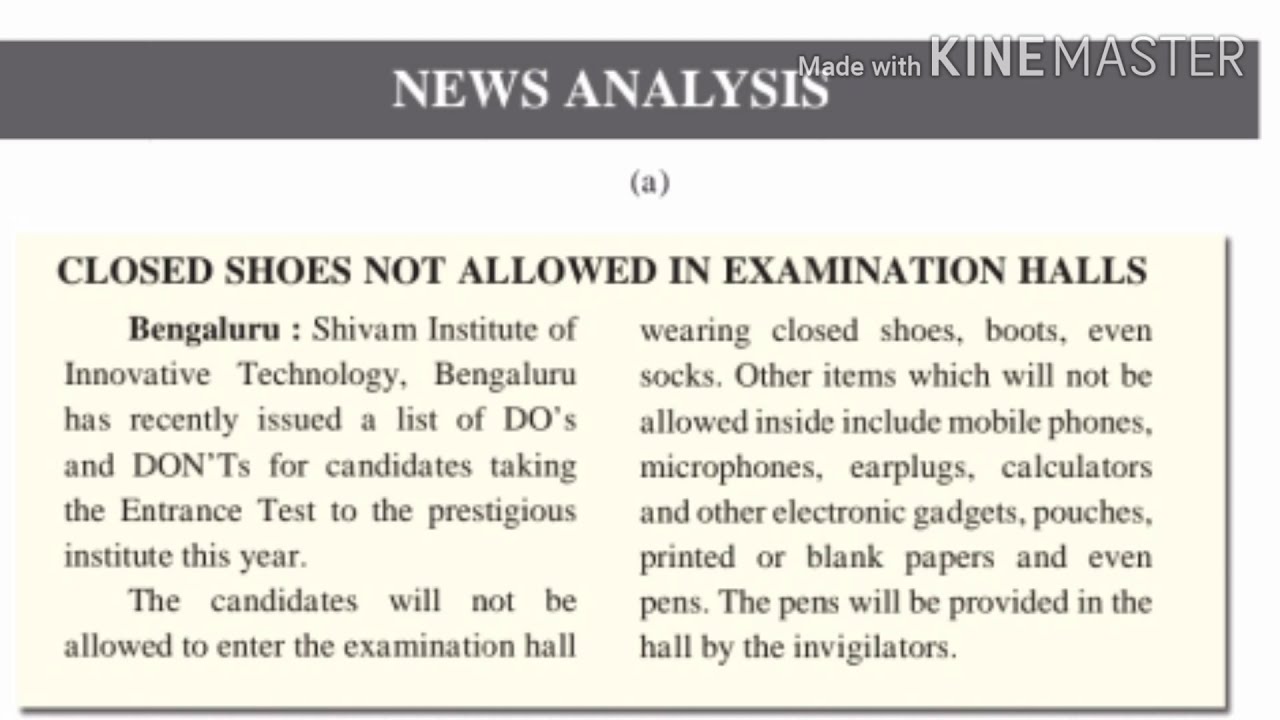The image is a close-up screenshot of a news analysis article, likely a digital version. At the top, a gray rectangular bar with the white, all-caps text "NEWS ANALYSIS" serves as the header. In the upper right-hand corner, there is faded white text that reads, "Made with KineMaster," indicating the screen capture program used. Below the header, the main content is set against a beige, neutral background. The prominent title in bold black text reads, "Closed Shoes Not Allowed in Examination Halls." The text details the rules issued by the Bengaluru Shivam Institute of Innovative Technology for candidates taking the entrance test this year. It specifies that closed shoes, boots, even socks are not allowed in the examination hall. Additionally, prohibited items include mobile phones, microphones, earplugs, calculators, other electronic gadgets, pouches, printed or blank papers, and pens, the latter of which will be provided in the hall by invigilators. The text is organized into a few paragraphs, split into two sections. There is a small lowercase "a" in parentheses between the header and the main text block on a white background.